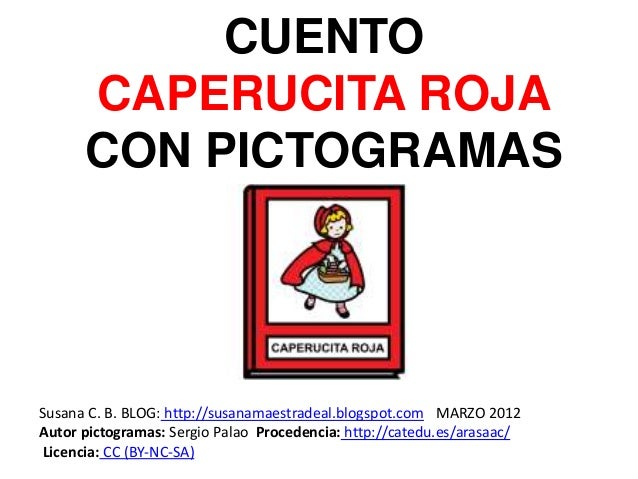The image features a predominantly white background with several lines of black and red text at the top. The first line says "Cuento" in large black letters, followed by "Capirusita Roja" in large red letters, and then "Con Pictograms" in large black letters, all in capital letters. Below this text is an illustration of a red book titled "Capirusita Roja." The book's cover depicts a cartoonish Little Red Riding Hood—a white girl with blonde hair wearing a red hooded cape and a blue and white dress, carrying a basket. The book appears to be framed by a white rectangle. Beneath the book, there is additional text: "Suzanne C.B. Blog," followed by the URL "http://suzannemaestredell.blogspot.com." Further below this is text attributed to "Author Pictograms Sergio Palo Prodeocea" and another URL "http://catedu.es/a-r-a-s-a-a-c/lacienza cc by n-c-s-a," which indicates the image is possibly related to educational resources or a blog post in Spanish from March 2012. The text layout occupies more space than the book illustration, with all text in black except for "Capirusita Roja," which is in red.